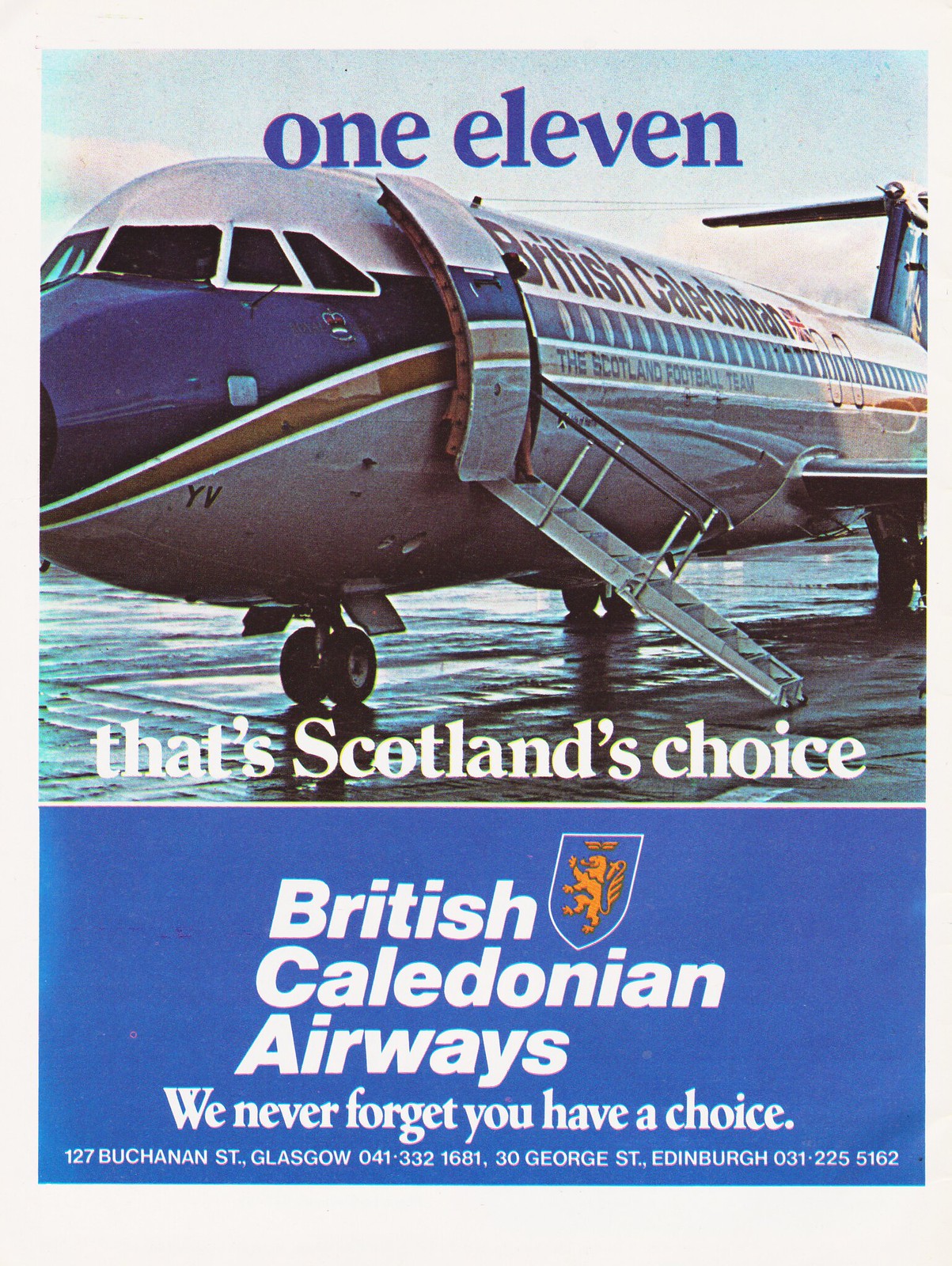This image appears to be a detailed advertisement for an airline, likely found in a magazine or a soccer program. The poster prominently features a photograph of a large commercial jet, seen from an angle where the front end is closer to the viewer than the rear. The aircraft, colored in a grayish silver with a distinctive blue stripe along the middle and nose, also features a red stripe running the length of its body and the text "British Caledonian" alongside the passenger windows. The door of the jet is open, with stairs leading up into it. 

At the top of the poster, dark blue text reads "1-11" followed by the phrase "That's Scotland's Choice," suggesting a connection to Scotland. Further supporting this, the jet bears the marking "Scotland football team," indicating it might be the team's designated transport. Below the airplane image, a blue text box prominently displays "British Caledonian Airways" in bold white text, alongside the company's slogan, "We never forget you have a choice." Adjacent to this, there's a shield-shaped logo with a crest-designed lion, reinforcing the Scottish theme.

Finally, the poster includes contact details at the bottom, listing addresses and phone numbers for British Caledonian Airways offices at 127 Buchanan Street, Glasgow, and 30 George Street, Edinburgh. The entire ad predominantly uses shades of blue, adding to its cohesive visual appeal.